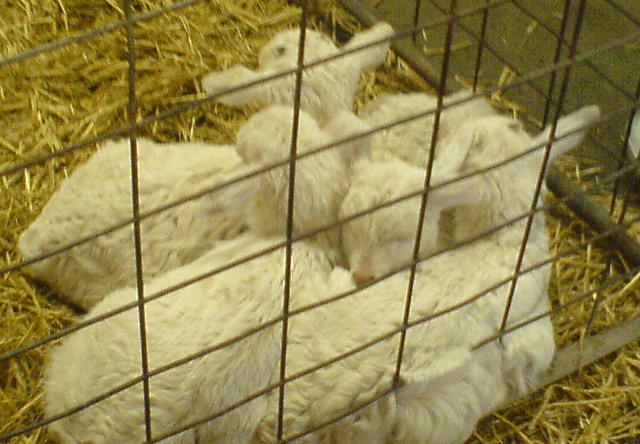This photograph captures a small wire holding pen containing four or five tiny, huddled baby lambs. The lambs are nestled into a bed of yellowish, golden straw that lines the bottom of the pen. The pen itself appears to be made of metal with wide spacing in the wire. Some of the lambs have their eyes closed, suggesting they might be sleeping. One lamb is distinctive with a little black spot on its head, while another has its fur sticking through the wire. The lamb closest to the fence has a pink nose, and all their ears are sticking straight out. The overall atmosphere is of peaceful rest in a small, contained space. Off to the side of the pen, there's a dark, grayish surface barely visible in the corner of the photo.